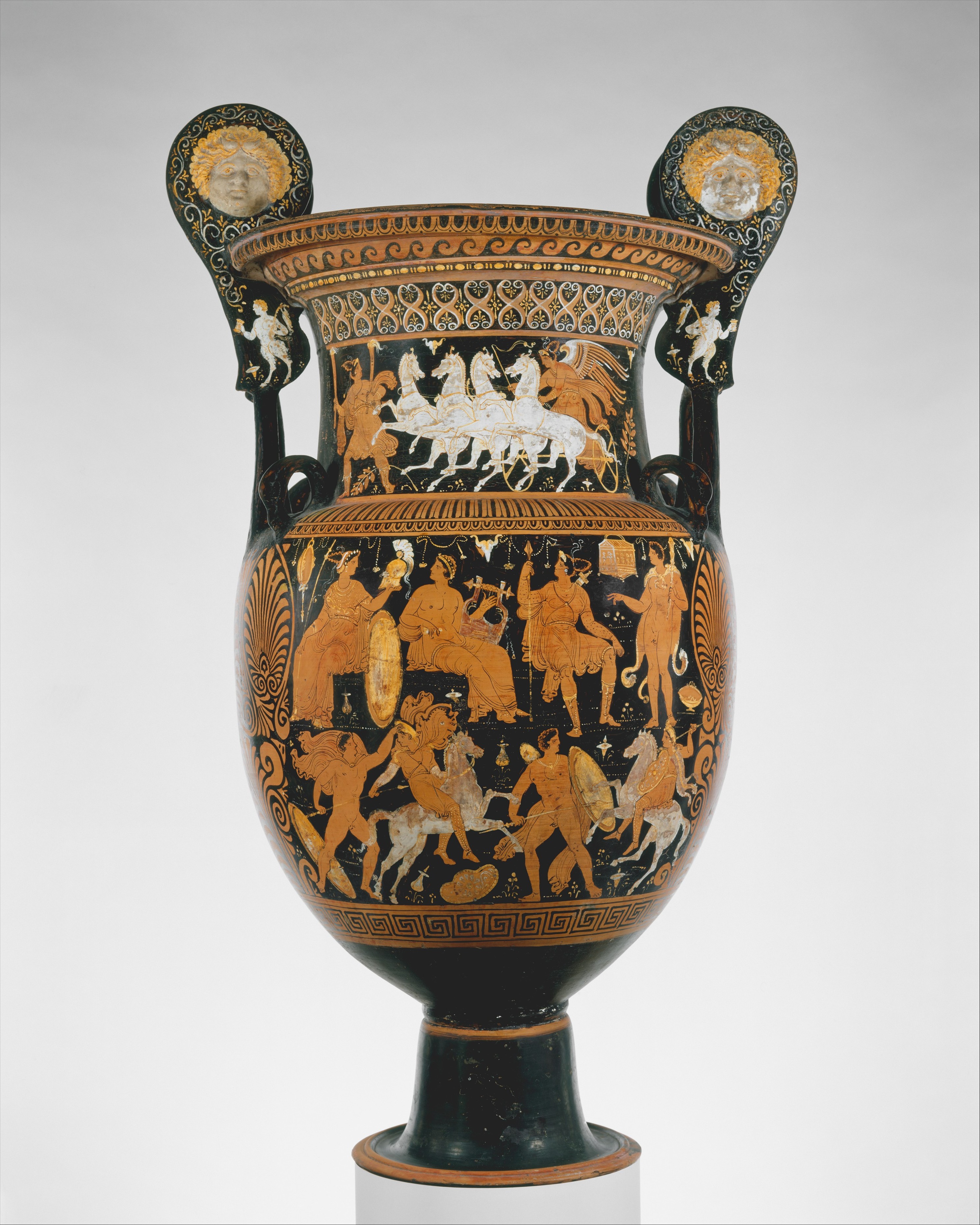This detailed image depicts a Grecian urn or vase, likely from the classical or archaic period. The primary color is black with a glossy finish, featuring intricate illustrations in dark gold or brown tones. The urn sits on a small circular pedestal base, which supports its bulbous center. The central portion is adorned with rows of human figures, including nude men and women, spanning across the breadth of the urn. Above these figures, there are additional illustrations including a chariot pulled by four white horses with a figure inside and a male figure to the left. This illustration is complemented by ornate wave patterns in a combination of black and orange.

The urn’s wide neck also features a band of detailed artwork, showcasing various mythological figures, some on horses and others possibly representing Greek gods, with some of these characters donning golden robes and carrying shields. At the very top, there is a circular rim, flanked by two handles that traverse from the bulbous base to attach again near the top, adorned with decorative elements, including cherub-like faces with blonde afros. These features are set against a gray-white background, which highlights the urn's classical elegance, almost resembling a large trophy.